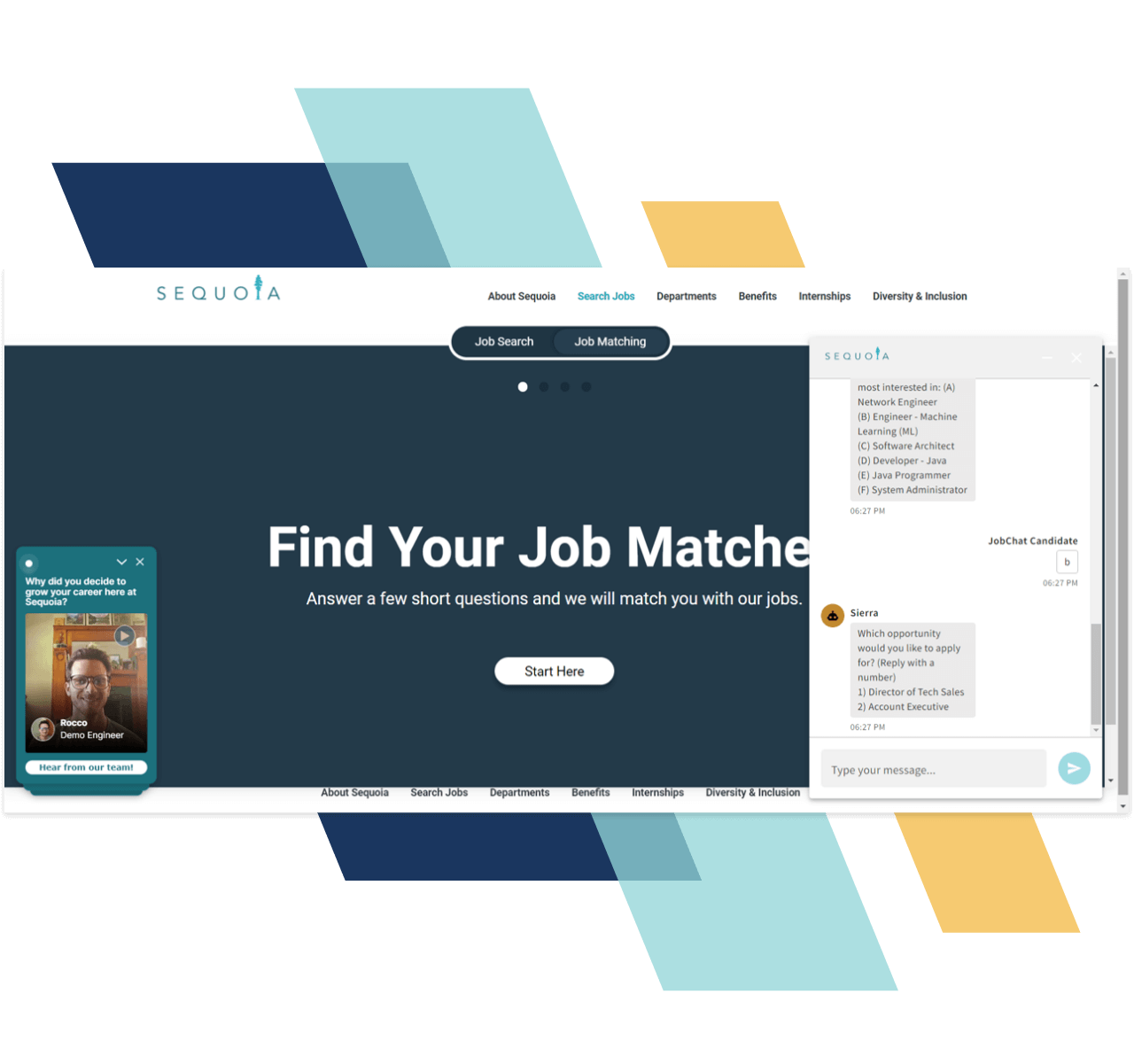Screenshot of Sequoia's Job Matching Page

The image is a detailed screenshot of Sequoia's online job search website. At the top left of the page, the company's name "Sequoia" is prominently displayed. Located in the navigation bar at the top of the page, there is an option labeled "Search Jobs" which has been clicked. The main feature of the webpage is a large, vibrant blue rectangle centered on the screen. Inside the rectangle, a headline states, "Find Your Job Matches," followed by the subtext, "Answer a few short questions and we will match you with our jobs."

Beneath this text, a prominent oval button labeled "Start Here" invites users to begin the process. In the bottom left corner of the blue rectangle, there appears to be an embedded video call screenshot. This image captures a smiling man with glasses and brown hair, identified as "Rocco, Demo Engineer," who is likely engaged in a video chat. The text above his image prompts with the question, "Why did you decide to grow your career here at Sequoia?"

On the right side of the screen, there is a white section resembling a chat interface. It features a message from "Sierra" asking, "Which opportunity would you like to apply for? Reply with a number." This is followed by job options: "1. Director of Tech Sales" and "2. Account Executive." At the bottom right corner of this chat section, a text box labeled "Type your message" allows users to respond.

Overall, the image details a user-friendly and interactive job matching interface provided by Sequoia, combining visual elements of video interaction with a straightforward question and answer format to help candidates find suitable job openings.